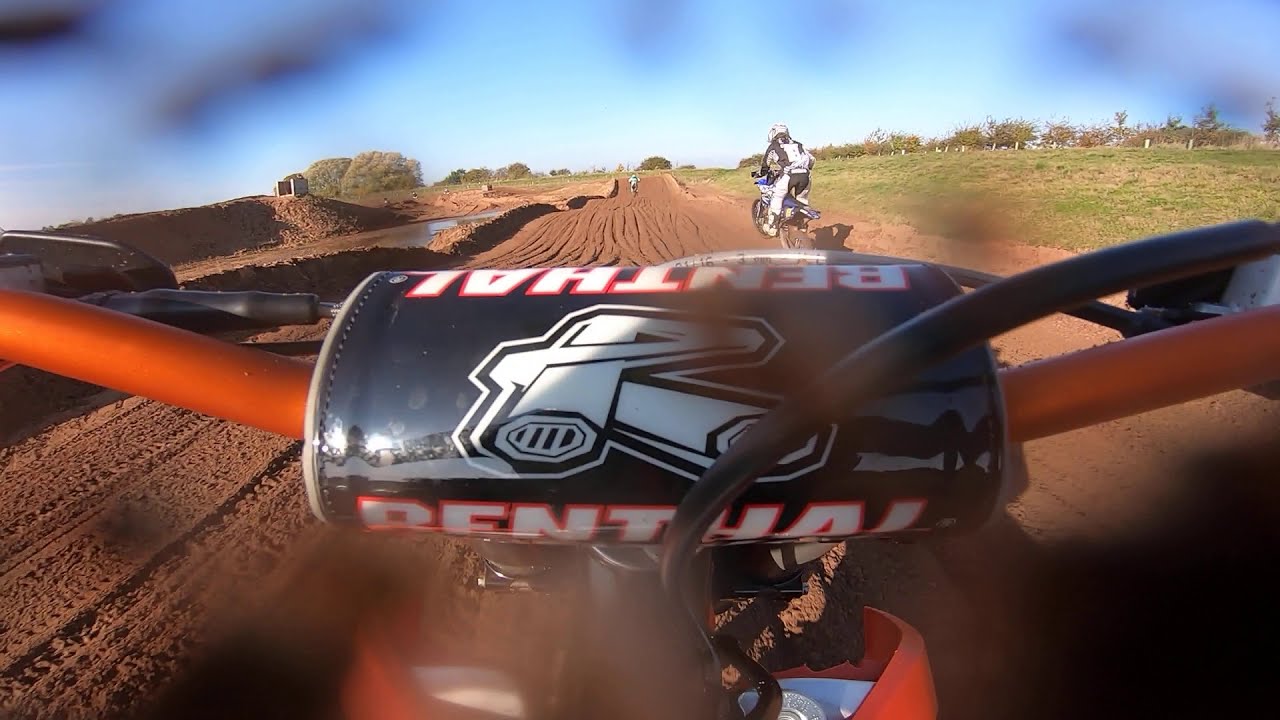The photograph, taken from the vantage point of a motorcycle mid-race, offers a captivating perspective right between the handlebars. The handlebars are adorned with orange grips and a protective pad, which prominently displays the logo "Renthal." Cables for the brakes and clutch snake through the center of the image, adding to the dynamic action captured. The dirt bike, featuring an orange gas tank, appears to be traversing a muddy, well-defined race track that extends vertically up the frame.

Ahead of this bike, two racers can be seen: one in the distance, possibly mid-jump, and another riding fast on the track. The clear blue sky, void of clouds, suggests a bright, sunny day perfect for outdoor racing. Flanking the track are patches of green field, enhancing the contrast with the brown dirt path. The overall scene, set against a stunning backdrop of natural colors—orange, black, red, white, green, brown, beige, tan, and light blue—depicts an exhilarating dirt bike race unfolding on an established track.